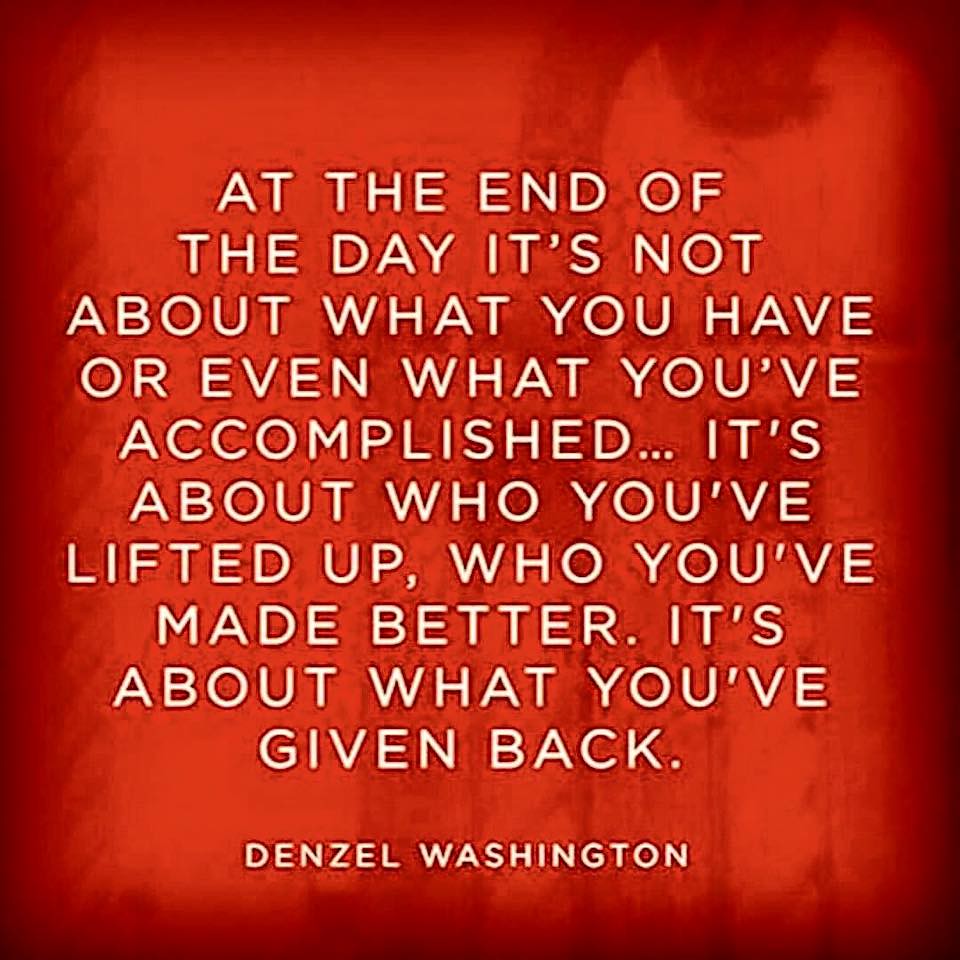The square image features a striking dark red background that transitions to black around the edges, with textured black shadows adding depth to the center. Against this rich backdrop, large white letters boldly display an inspirational quote: "At the end of the day, it's not about what you have or even what you've accomplished. It's about who you've lifted up, who you've made better. It's about what you've given back." Below the quote, in slightly smaller white letters, is the attribution, "Denzel Washington." The lower part of the image subtly lightens to an almost orange hue, creating a gradient effect that enhances the overall visual impact. The contrast between the dark red and the white lettering makes the message stand out, likely intended for social media to ensure it catches the eye and conveys its motivational message.